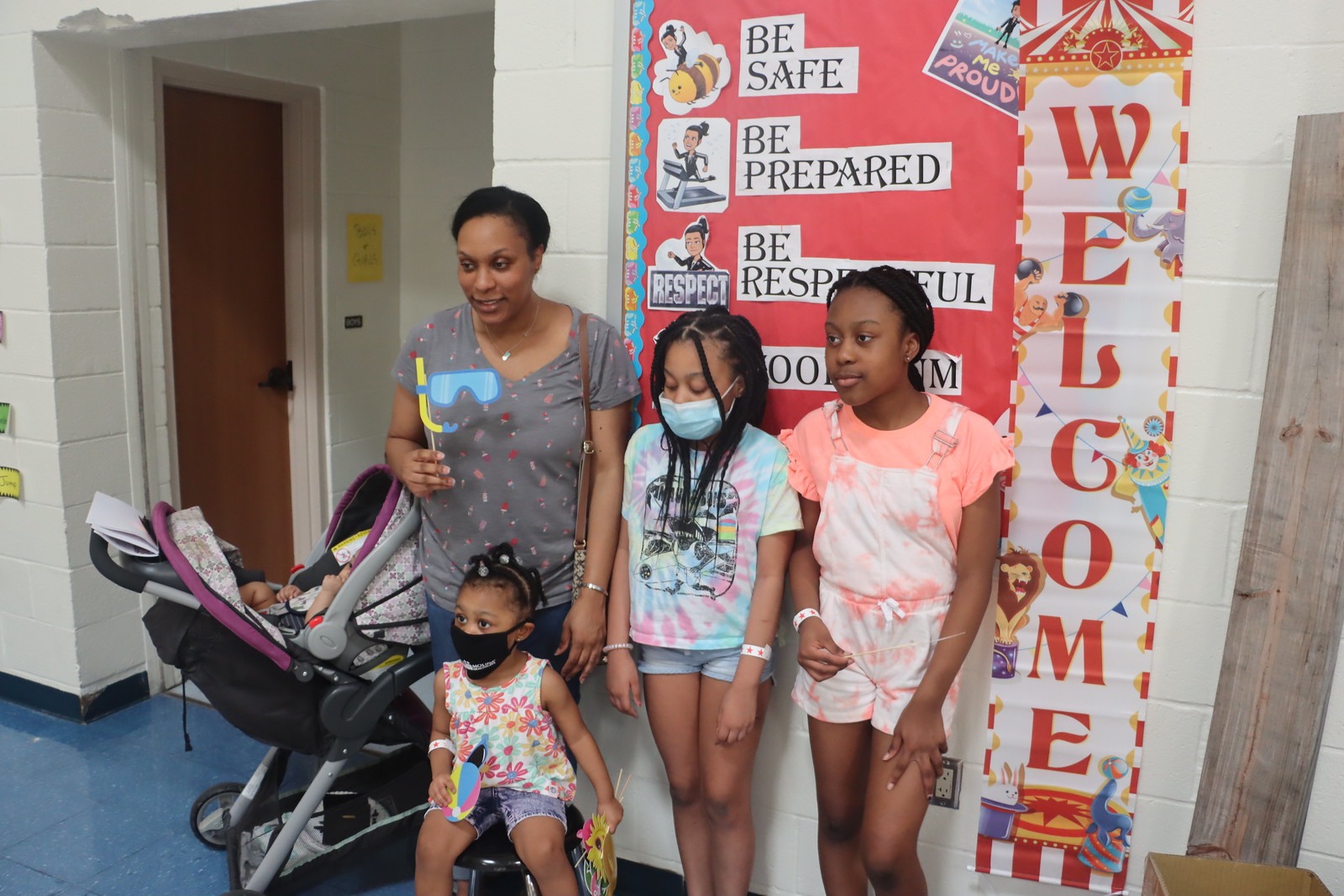An indoor photograph captures a Black family at what appears to be a school setting. The mother stands to the left of her four children, who seem to range in age from about 12 to 5 years old. Two of the daughters are wearing blue face masks. The youngest child is seated in a black stroller with purple accents, positioned behind the mother. They are all looking slightly to the right, likely toward the camera. The mother, dressed in a gray top and jeans, is holding something in her hand. The children are dressed in colorful t-shirts, with the oldest daughter donning a matching pants and top set. Behind them, on a white cement wall with a closed brown door in an alcove, hangs a construction paper sign that reads, "Be safe, be prepared, be respectful." The scene suggests they are waiting to enter somewhere, emphasizing a backdrop of safety and preparedness.